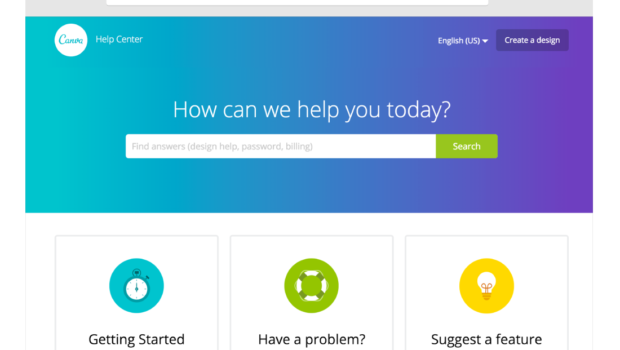On the website's Help Center page, the logo in the top-left corner is somewhat difficult to read. It features a white button with teal cursive writing, possibly starting with a 'C'. At the top of the page, there is a beautifully colored banner. It transitions from greenish teal to bluish teal and then to purple. Written in white lettering across this gradient is the phrase, "How can we help you today?" Below this text, there is a search bar where users can input queries such as "find answers", "design help", "passwords", and "billing suggestions".

Below the banner, the page background is predominantly white. There are three clickable rectangles aligned horizontally. The first one, labeled "Getting Started", features a picture of a stopwatch inside a teal circle. The second rectangle, titled "Have a Problem?", displays a green logo resembling a life preserver, but in green and white instead of the traditional red and white. The third rectangle, named "Suggest a Feature", has a yellow logo with a light bulb in the center.